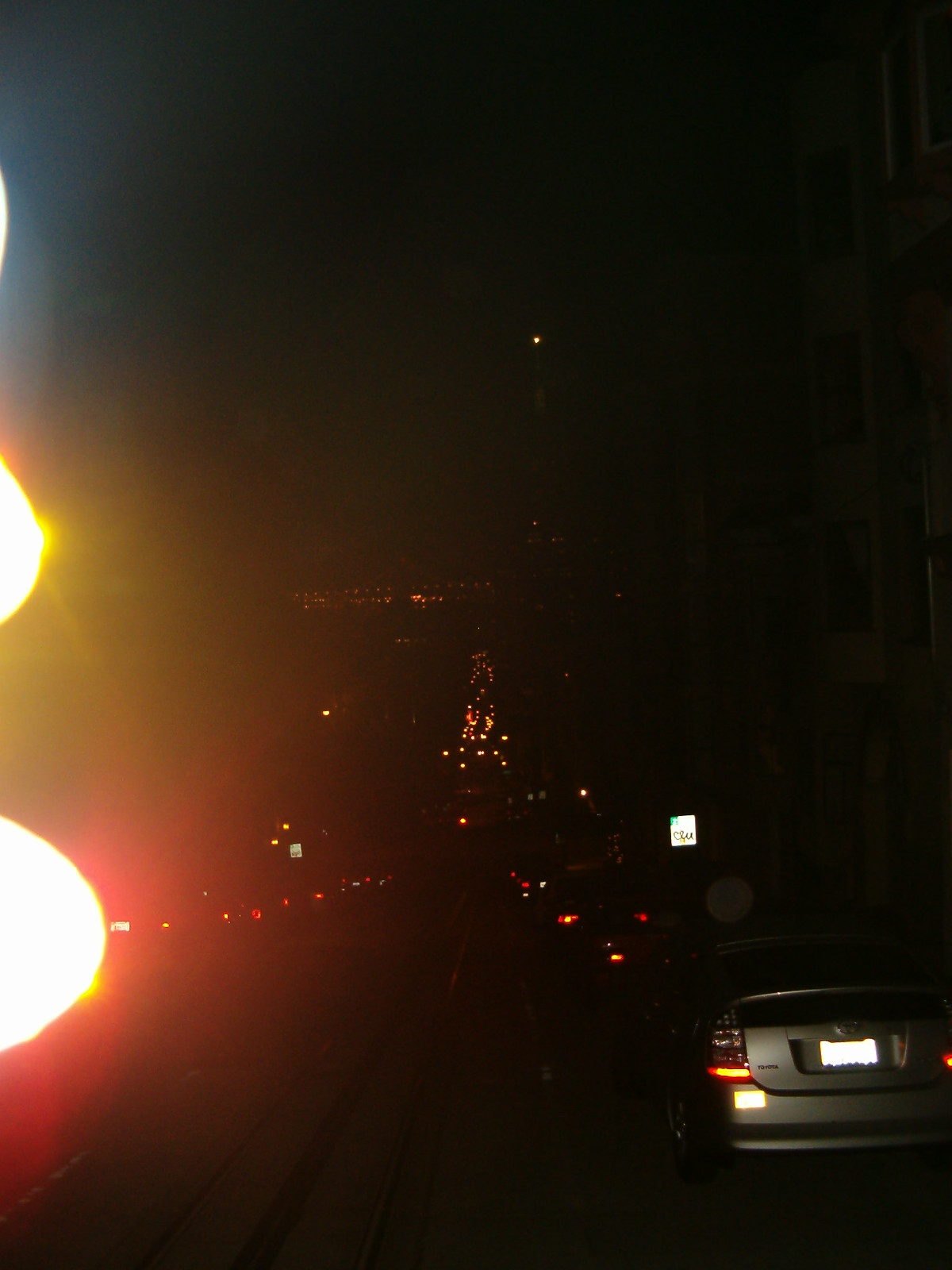This nighttime photograph captures an urban street scene illuminated by city lights and vehicle reflections. On the left side of the image, a yellow reflective surface partially appears, its source indistinguishable. On the right side of the street, a silver sedan is prominently seen in the foreground, while additional cars are visible further down the road. Street signs reflect the ambient light, contributing to the city's nighttime glow. In the background, city lights emit an amber radiance, and taillights from distant vehicles add a pop of red to the scene. Along the right edge, the outlines of buildings are discernible, including one predominantly white structure with visible windows. A subtle white lens flare effect enhances the photograph's dramatic nighttime ambiance.